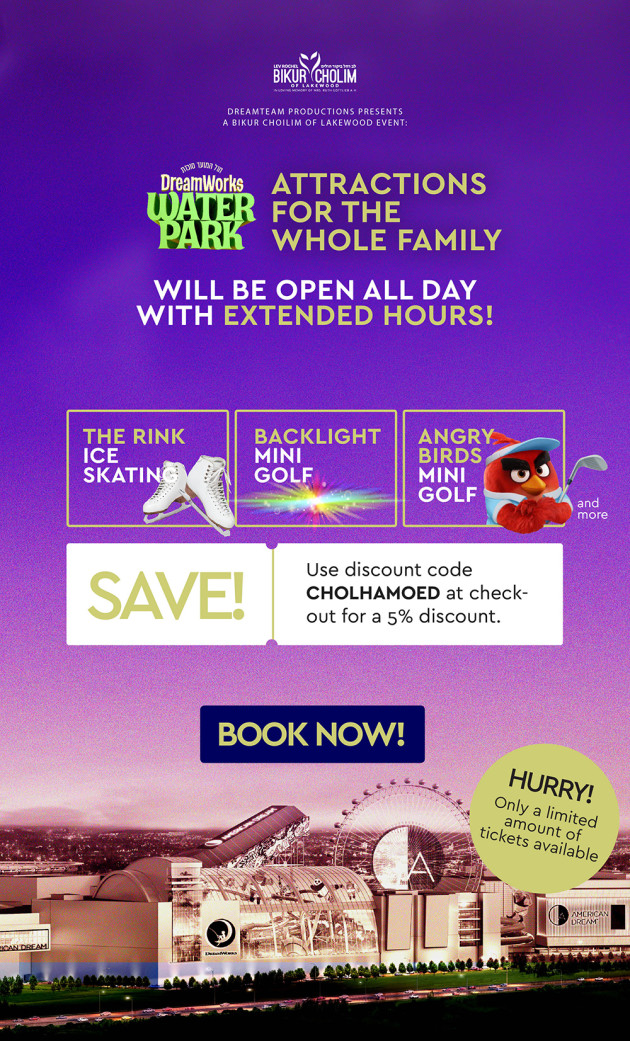**Advertisement for Bikur Cholim Event at DreamWorks Waterpark**

At the very top of this advertisement, the text reads “B-I-K-U-R-C-H-O-L-I-M.” Below, it states: "Dream Team Productions presents a Bikur Cholim of Lakewood event."

The headline announces: "DreamWorks Waterpark attractions for the whole family will be open all day with extended hours."

Three outlined green rectangles highlight specific attractions:
- The far-left rectangle features "The Rink Ice Skating."
- The middle rectangle promotes "Backlight Mini Golf."
- The far-right rectangle advertises "Angry Birds Mini Golf."

Additionally, there is a note saying: "and more."

Further down, a ticket-shaped rectangle provides discount information. On the left end, it reads "Save," and on the right end, it instructs users to "use discount code CHELLAMODE at checkout for a 5% discount."

Near the bottom center, there is a prominent "Book Now" button. Adjacent to it, a sticker-like label warns: "Hurry, only a limited amount of tickets available."